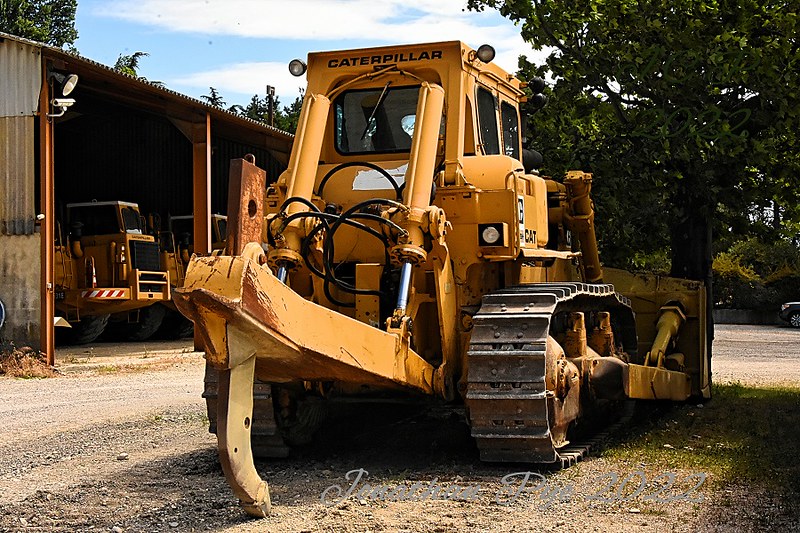A yellow Caterpillar bulldozer, branded with black lettering, is parked on a gravel road, facing away from the viewer. The machine's bucket is lowered to the ground and is positioned against a large green tree. To the left of the bulldozer stands a makeshift metal garage housing additional construction vehicles, one of which bears a red and white warning label. The garage is equipped with a large spotlight and a white rectangular security camera mounted directly beneath it, extending from a piece of wood. In the distance, numerous trees can be seen, enhancing the rural ambiance. On the right-hand side of the image, the front tire of an SUV is visible, parked in the shade beneath another large tree.